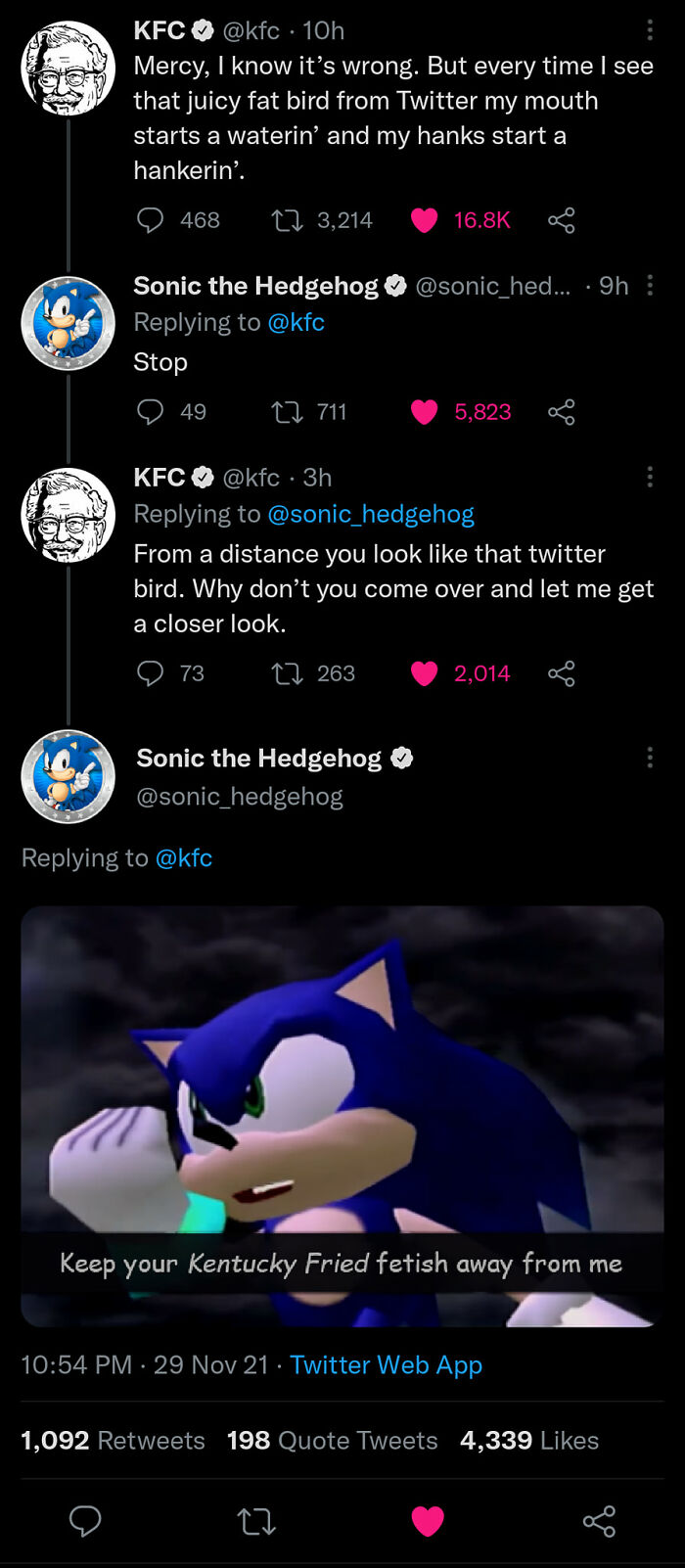Here is a detailed and cleaned-up caption for the image:

---

A screenshot of a humorous Twitter thread featuring a playful interaction between the official KFC account and Sonic the Hedgehog. 

1. **KFC (Handle: @KFC)**
   - **Profile Picture:** A black-and-white image of Colonel Sanders.
   - **Tweet:** "Mercy, I know it's wrong, but every time I see that juicy, fat bird from Twitter, my mouth starts watering and my hankering starts hankering."

2. **Sonic the Hedgehog (Reply):**
   - **Tweet:** "Stop."

3. **KFC (Reply to Sonic):**
   - **Tweet:** "From a distance, you look like that Twitter bird. Why don't you come over and let me get a closer look?"

4. **Sonic the Hedgehog (Final Reply with Image):**
   - **Image Description:** A picture of Sonic the Hedgehog with his fist up, looking towards the camera.
   - **Text Overlay on the Image:** "Keep your Kentucky Fried Fetish away from me."

---

This cleaned-up caption provides a clear and detailed description of the Twitter thread and the interaction between the two accounts.